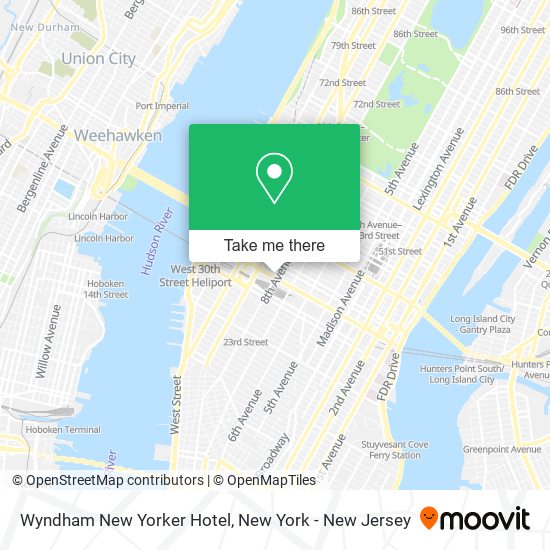This screenshot features a detailed map view of New York City, prominently displaying the location of the Wyndham New Yorker Hotel. The map is generated by the Moovit app, clearly noted by its logo "M-O-O-V-I-T" on the interface. The view is zoomed in, offering a comprehensive view of the urban landscape. To the left, the iconic Hudson River is visible, while an unlabeled body of water appears to the right. A highlighted marker pinpoints the exact location of the Wyndham New Yorker Hotel, and a pop-up window showcases a photograph of the hotel, providing a visual reference. This map aids in navigating the city and locating the hotel with ease.